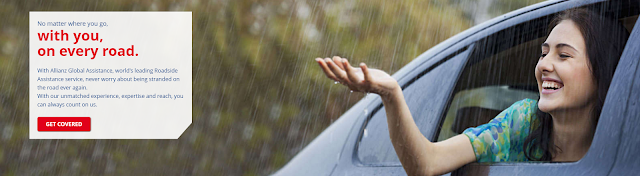In this landscape-oriented advertisement, the primary focus lies on a rain-streaked scene that transitions from the upper left to the lower left, where blurred raindrops cascade, creating a sense of heavy rainfall. Toward the center-right of the image, a light-skinned woman is captured in the passenger seat of a blue car. She beams with joy, her partially closed eyes and outstretched right arm welcoming the rain. Her green and light blue blouse is saturated with rainwater, which splashes off her open hand, illustrating her enjoyment of the moment.

The car's sleek blue exterior is partially visible, with the back window faintly noticeable amid the rainfall. On the left side of the image, a digital card prominently displays text. In bold, it reads: "No matter where you go," followed by "With you on every road" in striking red. Beneath, a slightly obscured message from Allianz Global Assistance promises world-leading roadside assistance services. The text assures, "Never worry about being stranded on the road ever again. With our unmatched experience, something in reach you can always count on." A noticeable blue button at the end encourages viewers to "Get Covered."

This vivid scene and reassuring message encapsulate the essence of the Allianz Global Assistance advertisement, showcasing their reliable service even in the most unexpected situations, as personified by the woman's carefree smile amidst the rain.